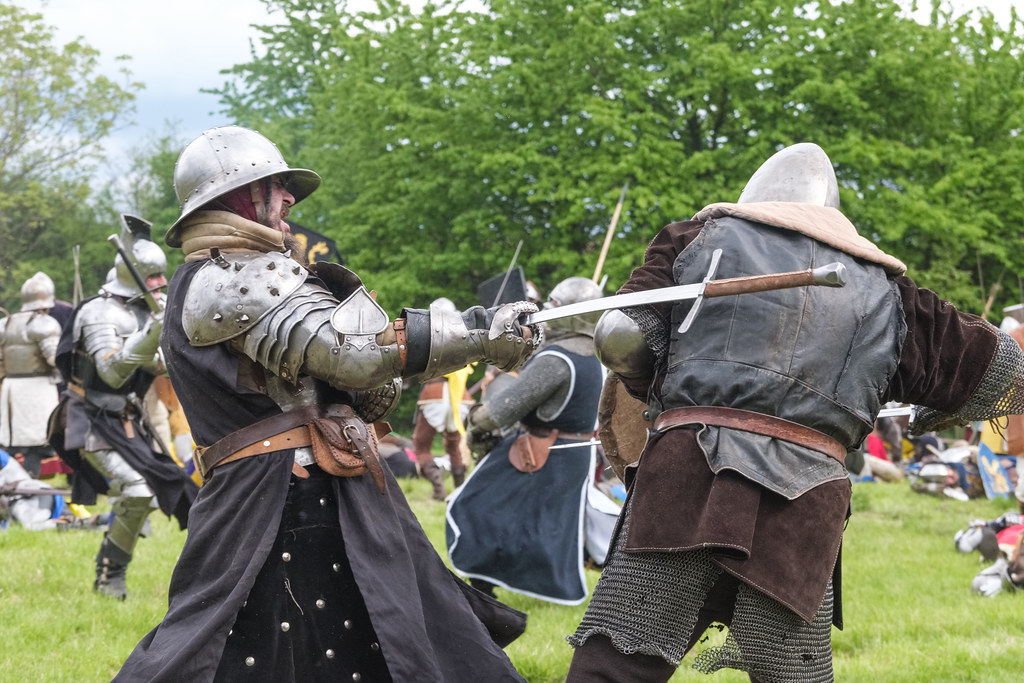In this captivating photograph of a historical reenactment, a lively scene unfolds in a lush, grassy field bordered by tall, green-leaved trees. Centered in the image are two men engaged in a mock battle, their outfits richly detailed and evocative of medieval times. The man on the left sports a rounded silver helmet, a black or gray cloak, and visible shoulder and forearm armor; he's grasping the blade of his sword, using the hilt to strike his opponent. The man to his right, facing away from the camera, wears a conical metal helmet and a gray tunic with dark brown sleeves, detailed with netting at the cuffs, over a long brown garment that extends below his waist, with chainmail visible underneath. In the background, numerous other participants dressed as knights wielding toy swords and shields can be seen in various stages of combat, evoking a spirited atmosphere of a Renaissance fair or historical role-playing event. The distant trees and expansive sky add a picturesque backdrop to this energetic, staged sword-fighting demonstration.